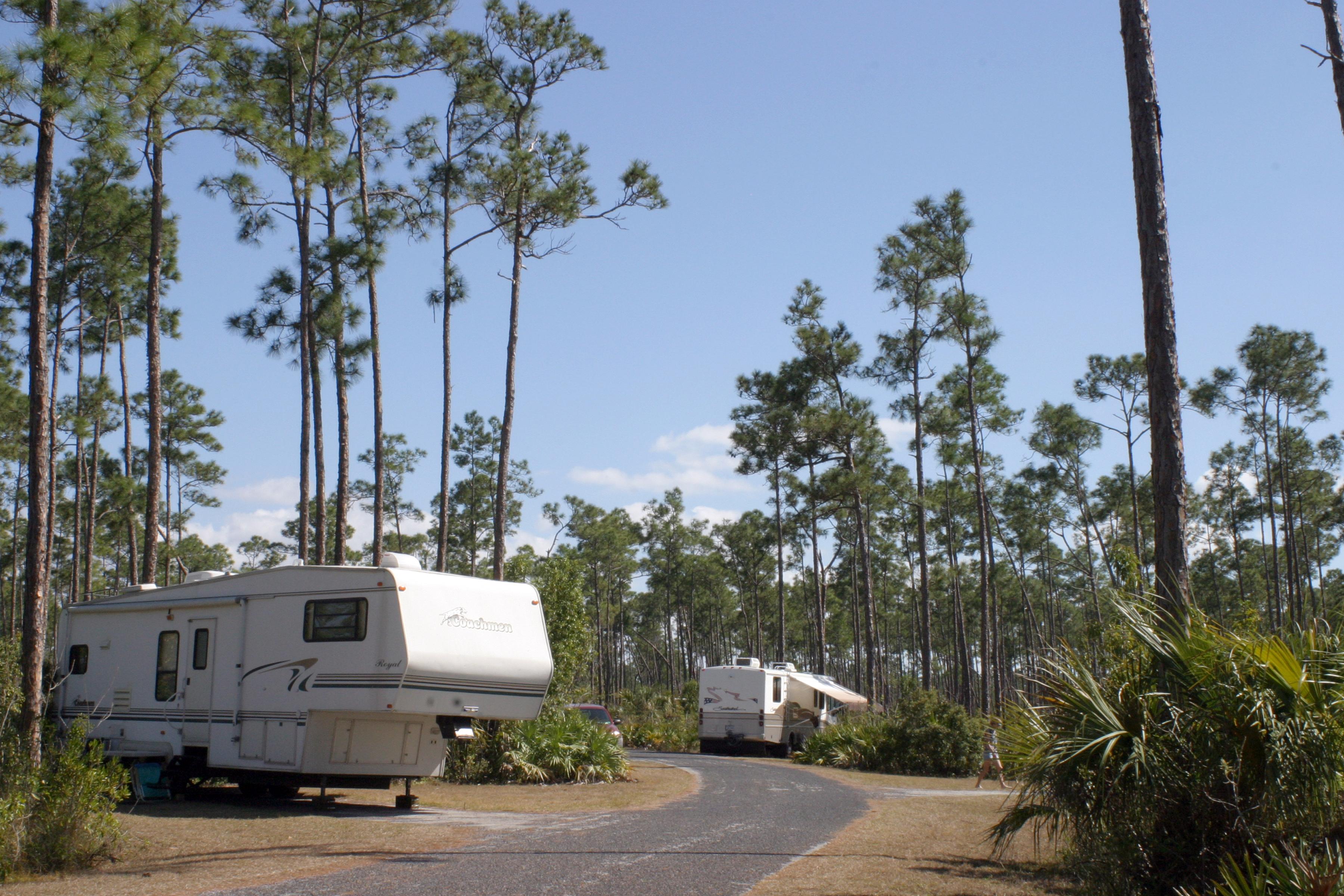The image depicts an outdoor campground scene under a clear blue sky with a few clouds. The landscape is dominated by very tall, thin trees that reach high into the sky, with most of their green foliage concentrated at the top, giving them a somewhat tropical appearance. In the foreground, there are two white RVs positioned along a narrow, curving road. The RV on the left is closer to the camera, partially blocking the view of the second RV in the middle of the image, which features a brown stripe about a fourth of the way up from the bottom. The second RV, further back in the frame, has an overhang or veranda for shade on its side. The ground consists of brown dirt or dried grass, and there are various plants and bushes around the bases of the trees, adding to the verdant feel of the setting. Additionally, a person can be seen walking off to the right side of the image.